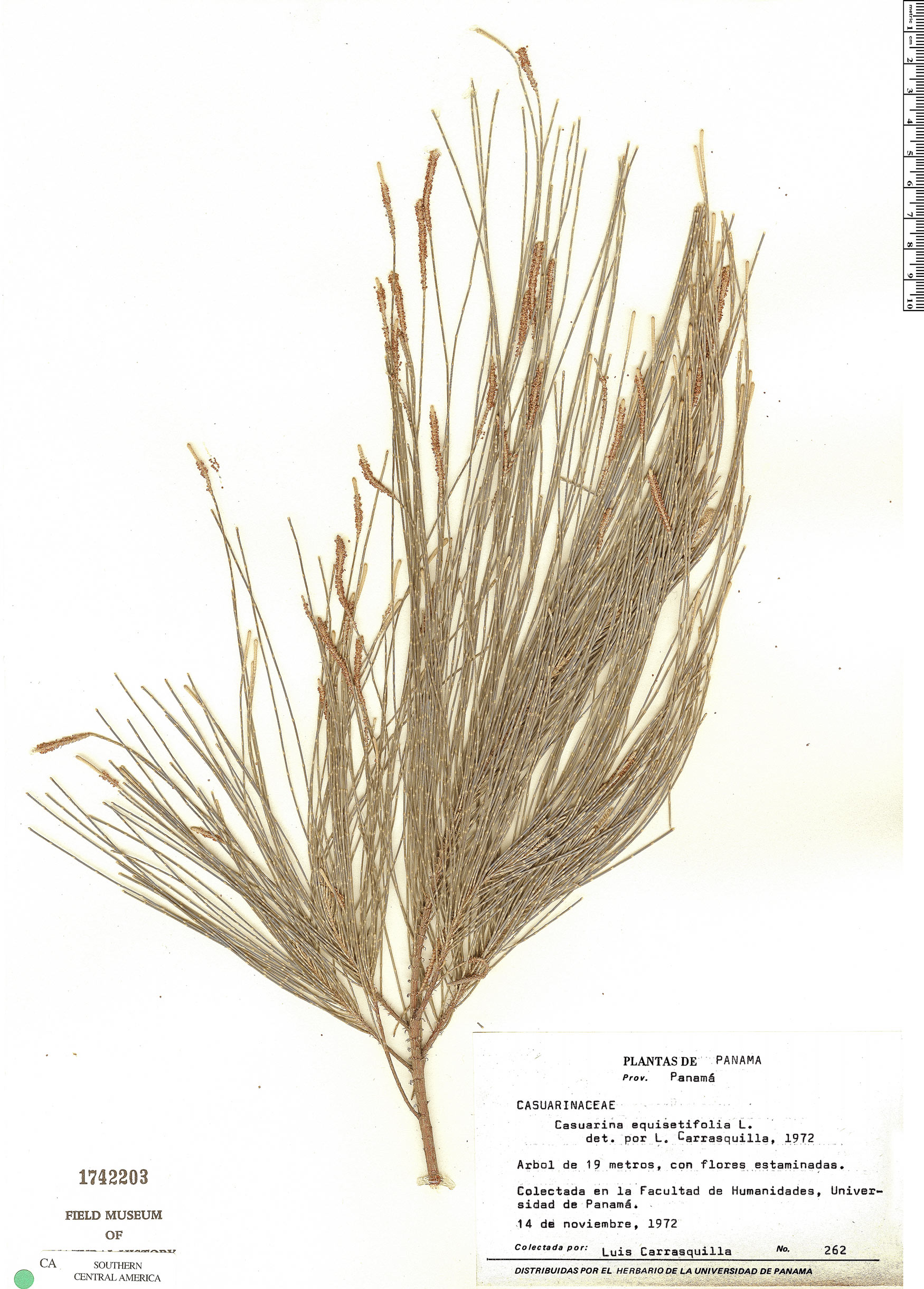This is a detailed scan of what appears to be a part of a plant belonging to the Casuarinaceae family, specifically labeled as Casuarina equisetifolia L. The image shows a brown twig adorned with thin, brown shoots and buds, presented like a museum exhibit. At the bottom right of the image, there is text in another language stating "Plantis De Panama" and "Universidad De Panama," suggesting the plant was collected or documented by the University of Panama. The bottom left of the display includes a label that reads "Field Museum of Southern Central America," accompanied by an item number "174-2203" and a green dot. A typewritten card with identifying information is also visible, indicating the specimen's classification and documentation date of 1972.